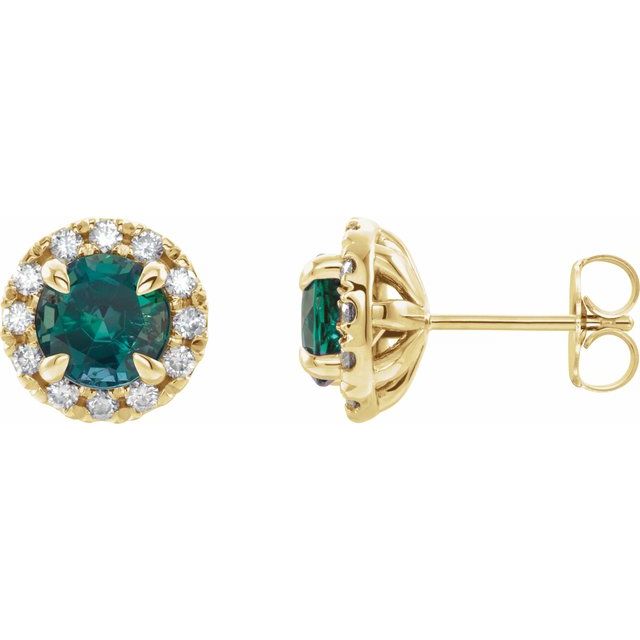This photograph is a high-resolution close-up showcasing a single stud earring with views from both the front and the side. Situated on a solid white background, the left side of the image features a top-down perspective, displaying a circular green gemstone, possibly an emerald, encased in a gold frame surrounded by a ring of sparkling white diamonds. The right side captures the side profile of the earring, revealing a gold stem that extends to a curved clasp, designed to secure the earring through the ear. The meticulous design showcases the intricate details, such as the alternating diamonds and the sturdy gold setting, making it a perfect image for a catalog or online sales listing.